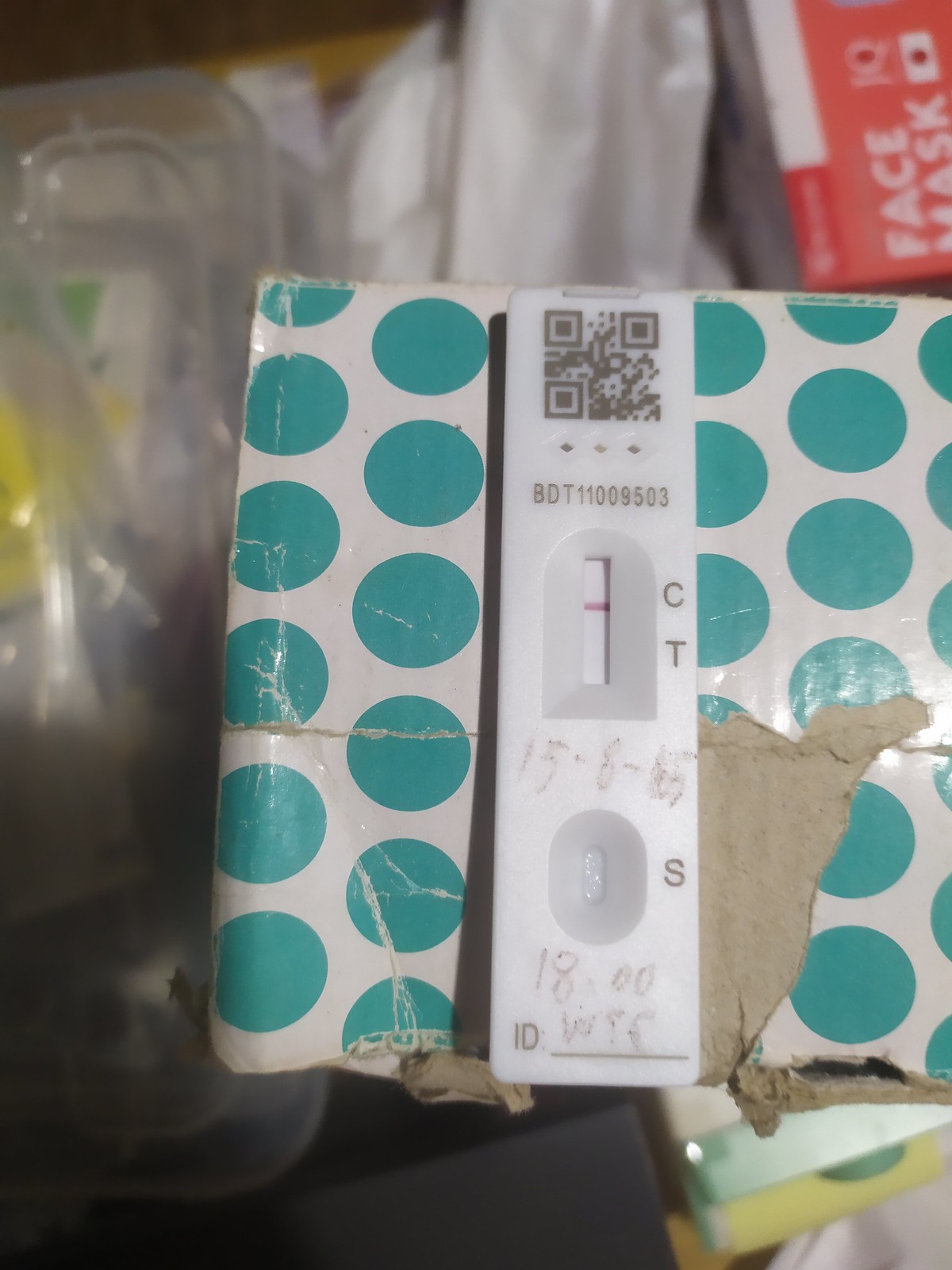The image features a COVID-19 test placed on a white box patterned with blue or turquoise polka dots, possibly a tissue box. The surrounding environment is cluttered, with plastic boxes, bags, and a red box labeled "face mask" visible but out of focus in the background. The COVID-19 test itself is a long, white rectangular stick displaying a QR code at the top, followed by the numbers "BDT 11009503". The test strip has a bar labeled "CT" with a red line across it. Additionally, the numbers "15, 8," and an indistinguishable final digit, likely representing a date, are written on the test. Below this, there is an area marked for dropping the test fluid, labeled with the time "1800". The section labeled "ID" shows handwritten characters that appear to read "WTF" or something similar.